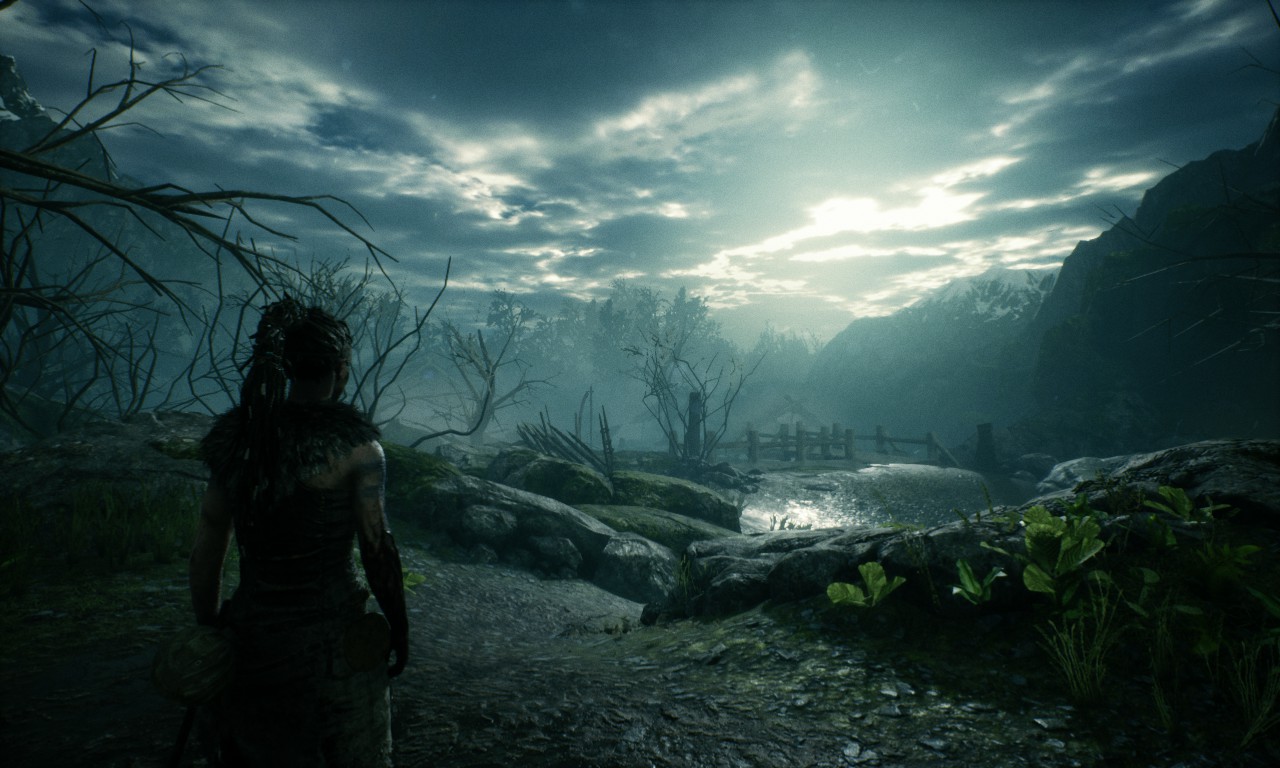In this horizontally rectangular, computer-generated fantasy scene, the viewer’s perspective is anchored by a lone figure in the lower left side of the frame. This person, who has their back to the viewer, is depicted from just above the knees upwards, with a ponytail cascading down their back. The ground beneath them is dark and subtly textured, providing a stark contrast to the rest of the scene. Directly in front of the figure lies an arrangement of rocks that slope downward toward the center before rising on the right, creating a natural barrier between the foreground and the expanse beyond.

Stretching from left to right along the middle of the image is a serene body of water, its tranquil surface a mirror to the dynamic sky above. Beyond the water, a lush landscape of trees and bushes melds seamlessly into a backdrop of towering mountains, adding layers of depth and mystery. Dominating the upper portion of the image, the sky is a spectacle of thick, dense clouds, casting an ethereal mood over the scene. Sunlight pierces through gaps in the cloud cover, illuminating the landscape with dramatic beams of light, giving the impression of a world caught between shadow and brilliance.